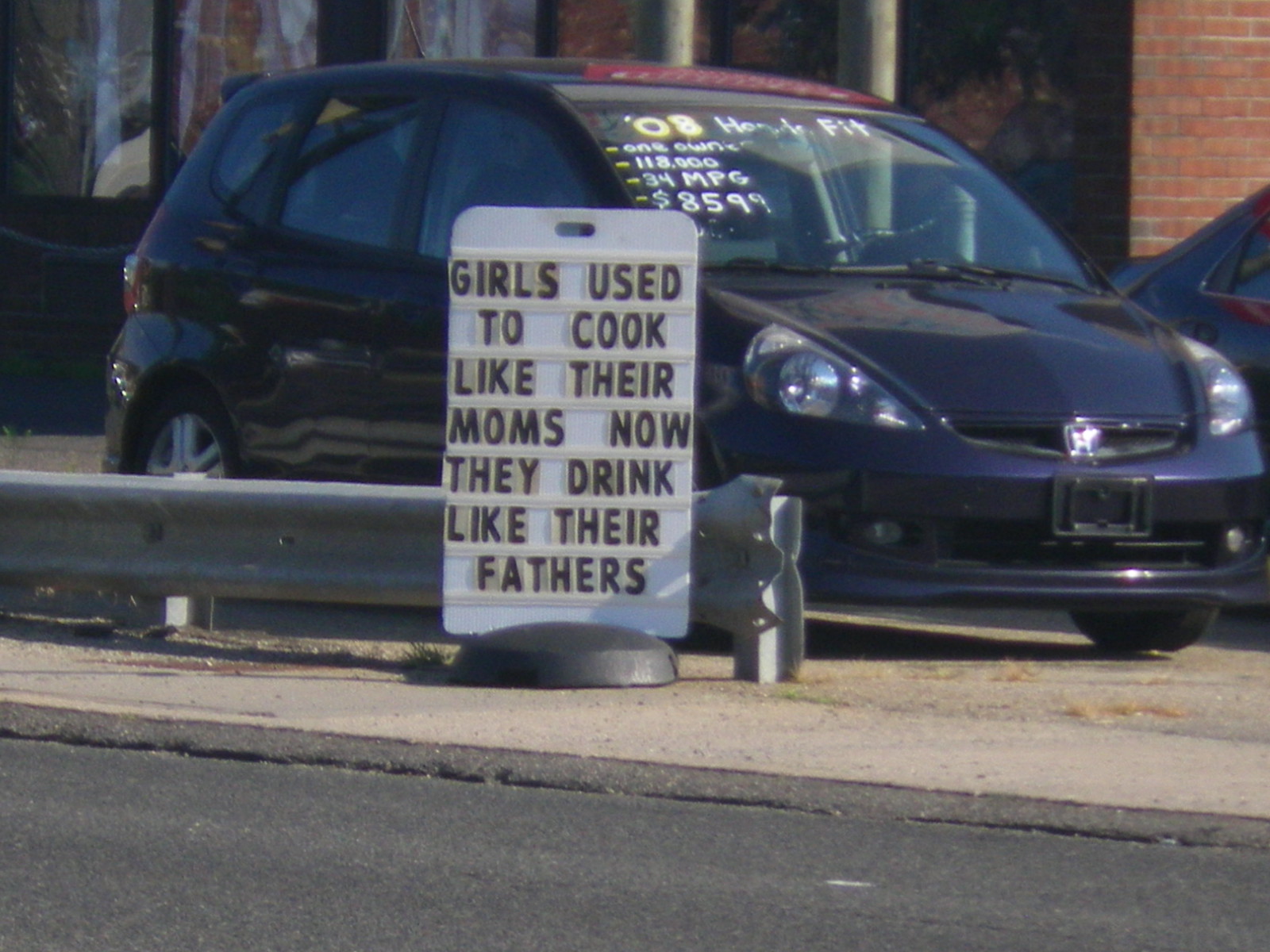In the image, a small van, which is actually a 2008 Honda Fit, prominently stands in a sales lot. This compact car, with its subcompact proportions and minivan-like silhouette, is priced at $8,599 as indicated on the windshield. The Honda Fit, known for its hatchback design, is nestled behind a notable signboard. This signboard, equipped with movable letters, humorously declares, "Girls used to cook like their moms. Now they drink like their fathers." The setting is further detailed with a guardrail in the foreground, accompanied by a narrow sidewalk and a visible stretch of the street beneath, creating a typical urban sales lot scene.